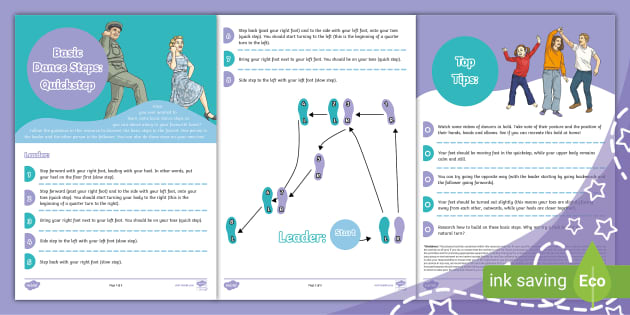The image appears to be an educational pamphlet, designed to teach basic dance steps. The background is primarily white and blue, with a purple border framing the entire page. In the top right corner, three people are seen dancing: two adults paired together, and a smaller child to their left. On the far left, two older individuals are shown dancing, seemingly performing the quick step. The center of the image features detailed shoe prints, illustrating different dance styles and labeled footprints to guide proper foot placement. The text, though partially unreadable due to its small size, includes phrases such as "basic dance steps," "quick step," "leader," "start," "top tips," "ink saving," and "ego." Various colors are used throughout the image, including shades of white, lavender, bluish-green, gray, army green, red, blue, orange, and light green. The bottom right corner contains an image of a leaf. The overall style is digitally crafted, emphasizing its instructional purpose.